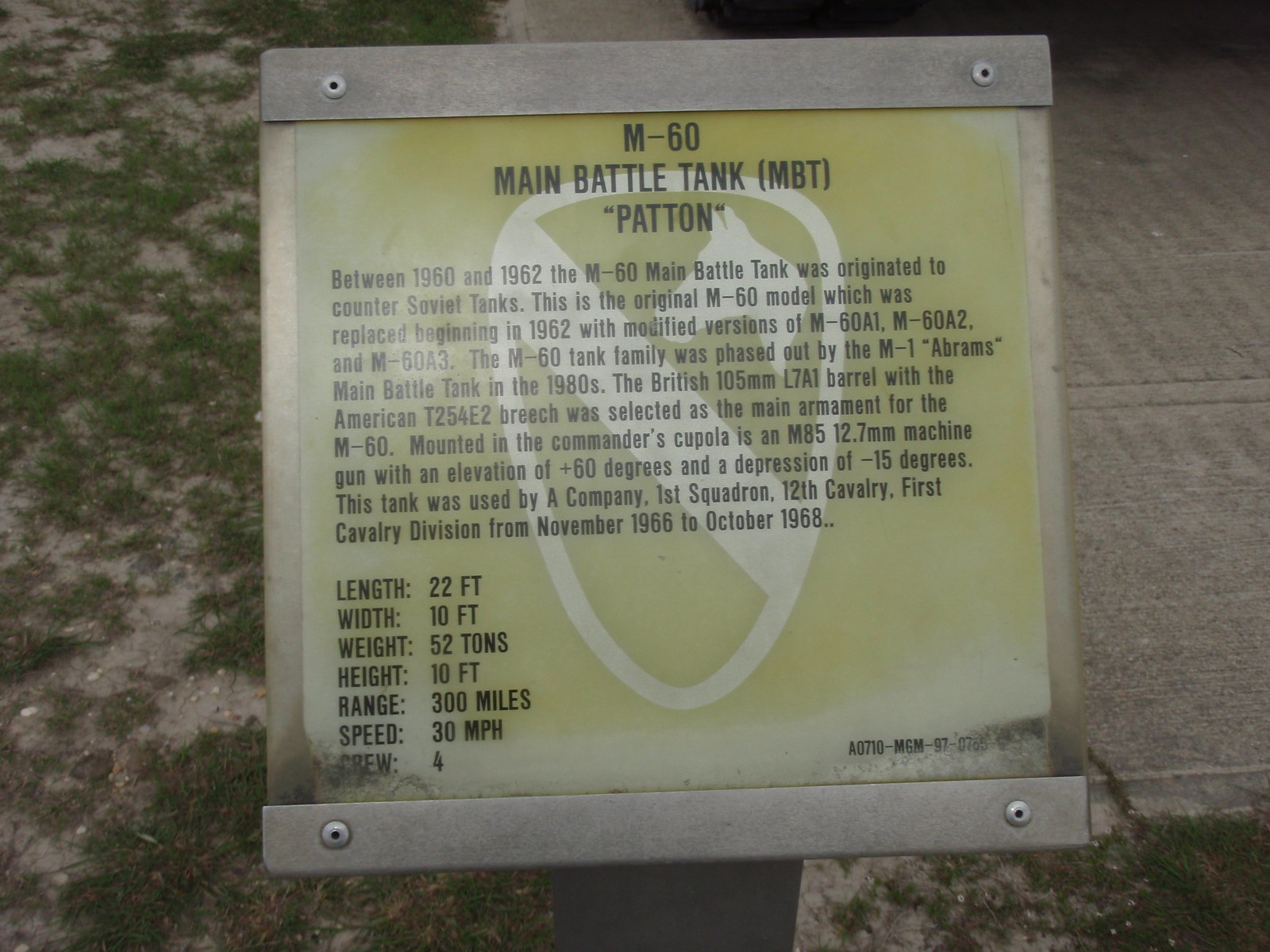The image depicts a green metal plaque, held up by two horizontal metal bars with screws at the ends, containing detailed information about the M60 Main Battle Tank, also known as the MBT Patton. The plaque is prominently adorned with the crest of the A Company, 1st Squadron, 2nd Cavalry, 1st Cavalry Division, featuring a shield with a diagonal slash and the outline of a dog's head on the upper right. The text on the plaque, written in black, covers the tank's history and specifications. The M60 was developed between 1960 and 1962 to counter Soviet tanks and used a British 105mm L7A1 barrel paired with an American T25-4E2 breech as its main armament. It also featured an M85 12.7mm machine gun mounted in the commander's cupola, with an elevation of 60 degrees and a depression of negative 15 degrees. This original M60 model was later replaced by modified versions (M60A1, M60A2, and M60A3) starting in 1962 and was eventually phased out by the M1 Abrams Main Battle Tank in the 1980s. The tank's dimensions include a length of 22 feet, a width of 10 feet, a height of 10 feet, and a weight of 52 tons. It had a range of 300 miles, a speed of 30 miles per hour, and accommodated a crew of four. The plaque's yellow background contrasts with the black text, making the information easily readable. The surrounding area in the photograph reveals a slightly grassy ground to the left and some asphalt or concrete to the right.